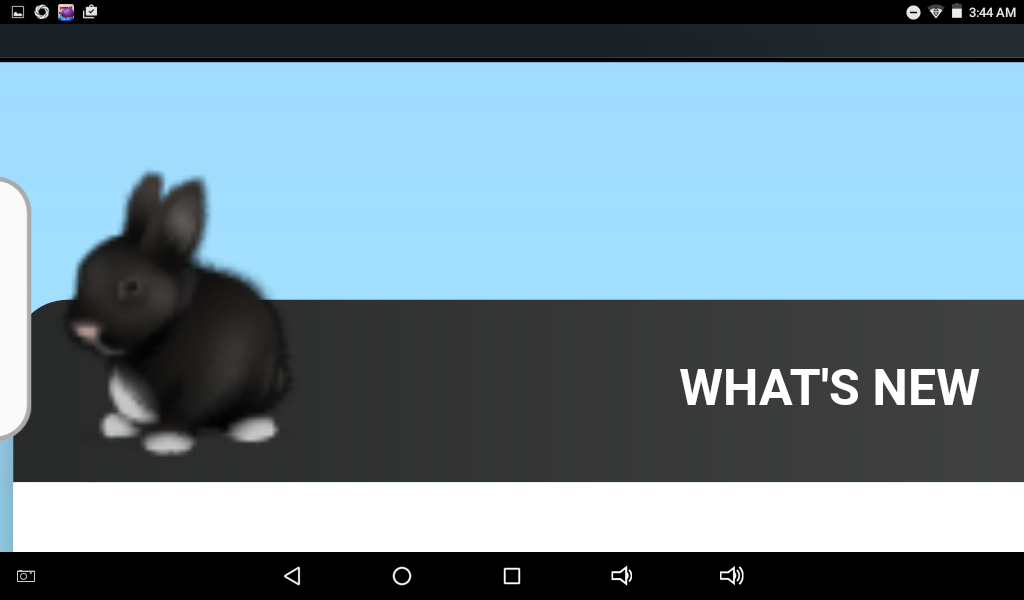This is a screenshot that appears to be from an electronic device, though it's difficult to discern whether it's from a smartphone or a computer due to its simple layout. At the top, there is a black header bar. On the left side of the header bar, there are four unfamiliar icons. On the right side, there are three icons, including a Wi-Fi connectivity icon, and the current time. 

Below the header, there is a prominent long blue rectangle, underneath which a long black rectangle is positioned. A black rabbit with white feet, a white nose, and a white mark on its chest overlaps these rectangles, with its body on the black rectangle and its head extending into the blue rectangle. 

To the right of the rabbit, bold, all-caps text reads "WHAT'S NEW." 

Further down, there is a white rectangle, followed by a black footer. The footer contains several icons: a camera icon, a back icon, a round home icon, a square overview icon, and two sound icons.